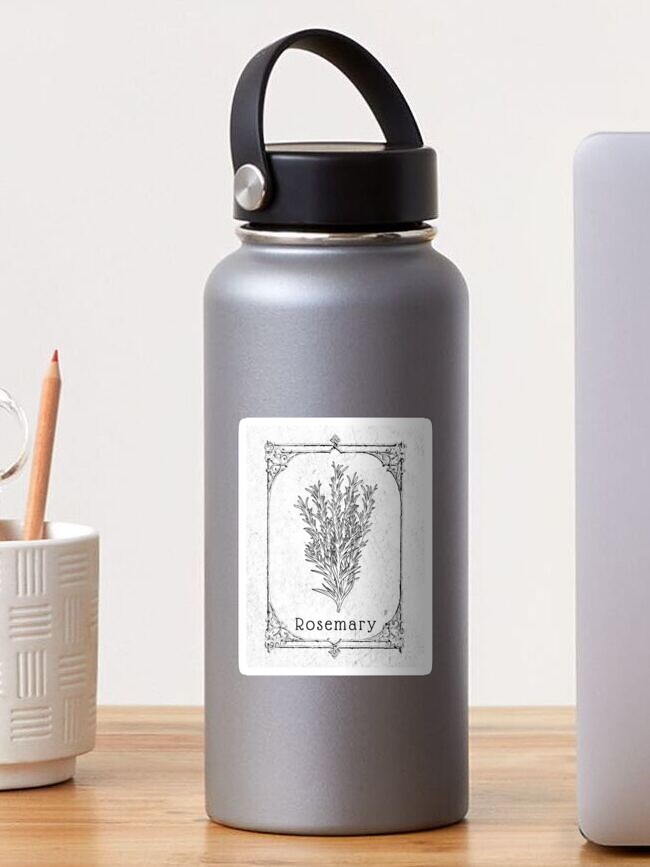In the image, there is a sleek, steel gray water bottle with a subtle shine, sitting on a medium-colored wooden desk. The water bottle features a black plastic top with a rubber handle looped from one end to the other, secured by two large metallic rivets. Separating the black plastic cap from the metal canister is a thin chrome metal lip. The bottle sports a white, rectangular label with a decorative border. Within this border is an illustrated plant, identified as "Rosemary" in clear text. To the left of the water bottle, sits a white ceramic cup holding a red-tipped colored pencil and a pair of metal scissors. On the right, partially visible, is the corner of a laptop, possibly a Mac. The backdrop is a plain white wall, and the water bottle, centrally placed, spans nearly the entire height of the image.